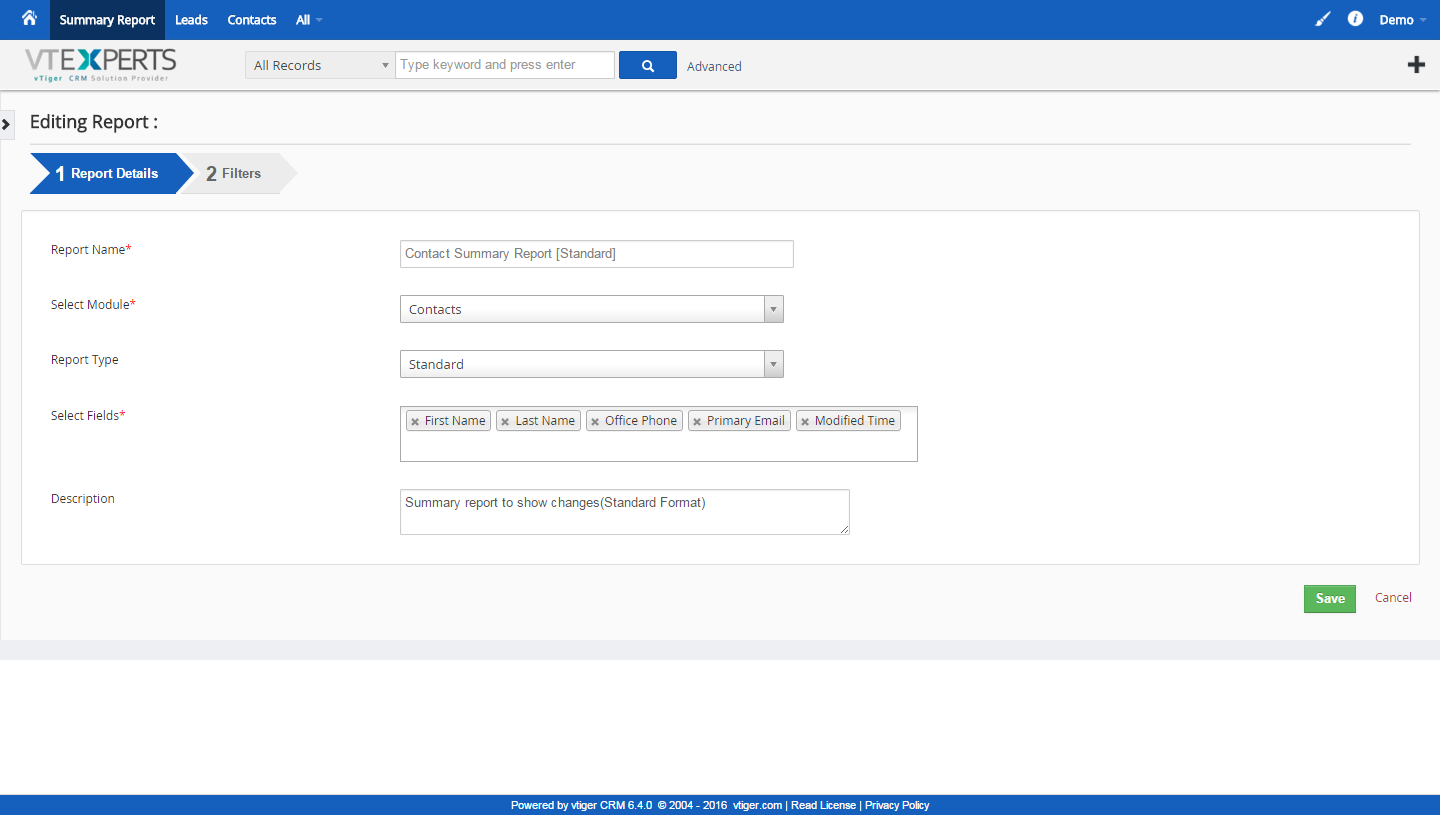This image is a detailed screenshot of the VT Experts website interface. At the top of the page, there is a blue banner featuring a white house icon symbolizing the home button, followed by navigation tabs labeled "Summary Report," "Leads," "Contacts," and an "All" drop-down menu. The current active tab is the "Summary Report."

The main body of the site is a light background, primarily white or light gray, showcasing the "Editing Report" section. This section is part of a two-step process, indicated by numbered steps at the top. The first step, "Report Details," is highlighted in blue, showing it is the current active step. The second step, "Filters," is shown in gray, indicating it is not yet active.

Within the "Report Details" step, there is a form to fill out, starting with an input box for the report name. Below this, you must select the appropriate module from a drop-down menu. Further options include selecting the report type from another drop-down menu, choosing relevant fields, and providing a description for the summary report.

All these inputs lead to the final action of saving the report by clicking the conspicuous green "Save" button located on the right-hand side of the form.

At the bottom of the page, another blue banner extends across the width of the screen, framing the website interface neatly. Due to the resolution, the text below "VT Experts" is too small to be legible.